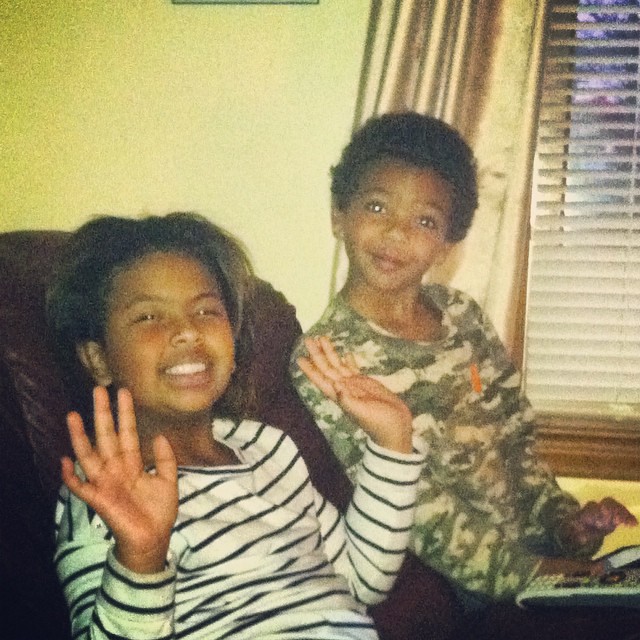In this endearing family photograph, likely taken in the late 80s or early 90s, two African descent children are positioned comfortably inside a warmly lit home with yellow walls. The girl, who appears to be anywhere between her teenage years to mid-twenties, sits on a brown recliner, dressed in a white long-sleeved shirt with black horizontal stripes. She is beaming with a full smile, her short brown hair framing her cheerful expression as she raises her hands up with open palms. To her right, a young boy, possibly between 7 and 10 years old, grins mischievously with his head slightly tilted. He dons a green and white camouflage long-sleeve top. Beside his right hand is a television remote resting on the recliner. The scene is completed with a metallic gold curtain and white blinds adorning a window in the background, giving the image an almost sepia-like nostalgic feel. The siblings look directly at the camera, capturing a moment of familial joy and connection.